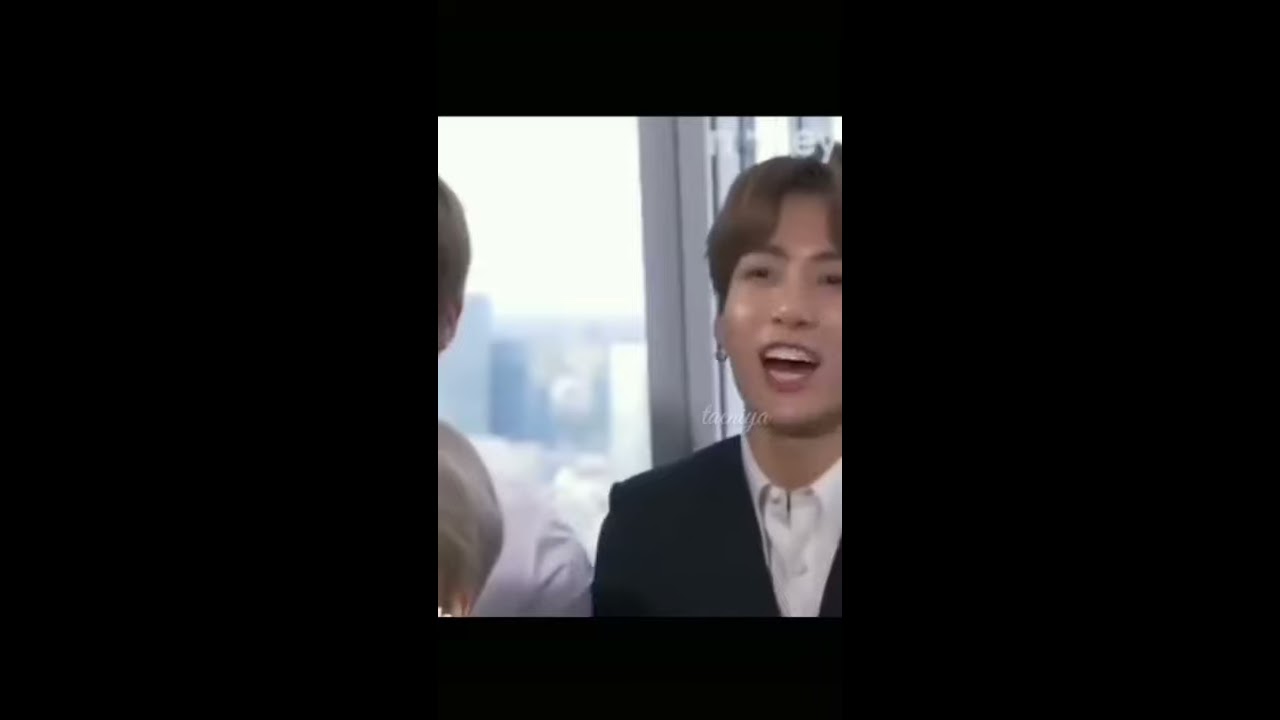This is a wide rectangular image where the background is completely black. In the center, there is a slightly tall rectangular photograph or screenshot capturing an energetic moment of an Asian man, partially cut off at the right edge of his eye. He has short to medium-length, dark blonde, swoopy hair parted in the middle and shiny, slightly tanned skin. The man, dressed in a white collared shirt with visible buttons and a dark suit jacket, is laughing heartily with his mouth open, revealing straight, white teeth and somewhat red lips. He appears to be standing or sitting in front of a slightly blurry cityscape visible through a gray window frame behind him. To the left edge of the image, you can glimpse parts of two heads or possibly the shoulder of another person, hinting at the man being in a social setting, perhaps reminiscent of an old-fashioned TV show. The overall scene suggests a lively, sunny day outside.